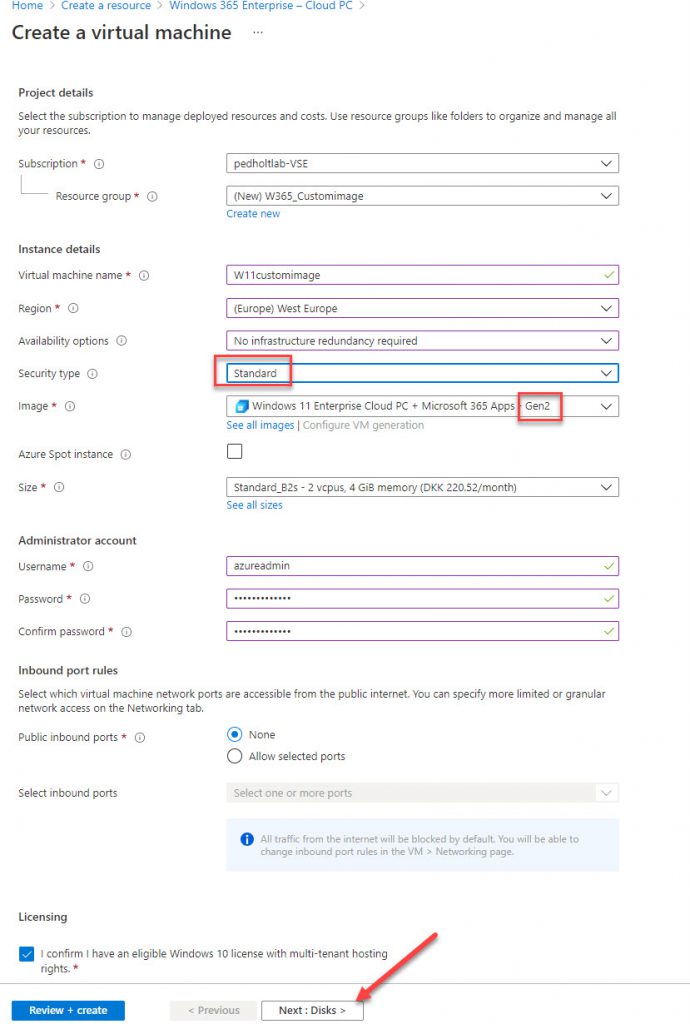This vertical image, resembling a computer screenshot, showcases a configuration interface for setting up a Windows 365 Enterprise - Cloud PC. The background is white, reflecting the computer screen’s default settings. 

At the top, a blue header bar displays the word "Home," followed by "Create a Resource: Windows 365 Enterprise - Cloud PC." Beneath this, aligned left in bold, is the heading "Create a Virtual Machine," followed by a smaller section titled "Project Details." This section continues with even smaller text explaining how to "Select the subscription to manage deployed resources and costs" and advises users to "Use resource groups like folders to organize and manage all your resources." 

Details provided in this part include the "Subscription" and associated resource group information, with an option to "Create New" via a blue button. Further down, under "Instance Details," it specifies the "Virtual Machine Name" and "Region," which is set to "West Europe." For "Availability Options," the choice is "No infrastructure redundancy required," and under "Security Type," "Standard" is selected. A red box highlights these options.

An "Image" section specifies "Windows 11 Enterprise Cloud PC Microsoft 365 Apps Gen 2," surrounded by another red box, with an option in blue to "See All Images" or configure additional settings. The form continues with sections for "Azure Spot Instance," "Size," "Administrator Account" with fields for username, password, and password confirmation, and "Inbound Port Rules," which shows "None" selected for public import ports. 

Finally, the interface offers a navigation bar with options for "Licensing," "Review + Create," and "Previous" or "Next." A red arrow points to the "Disks" section for further configuration.